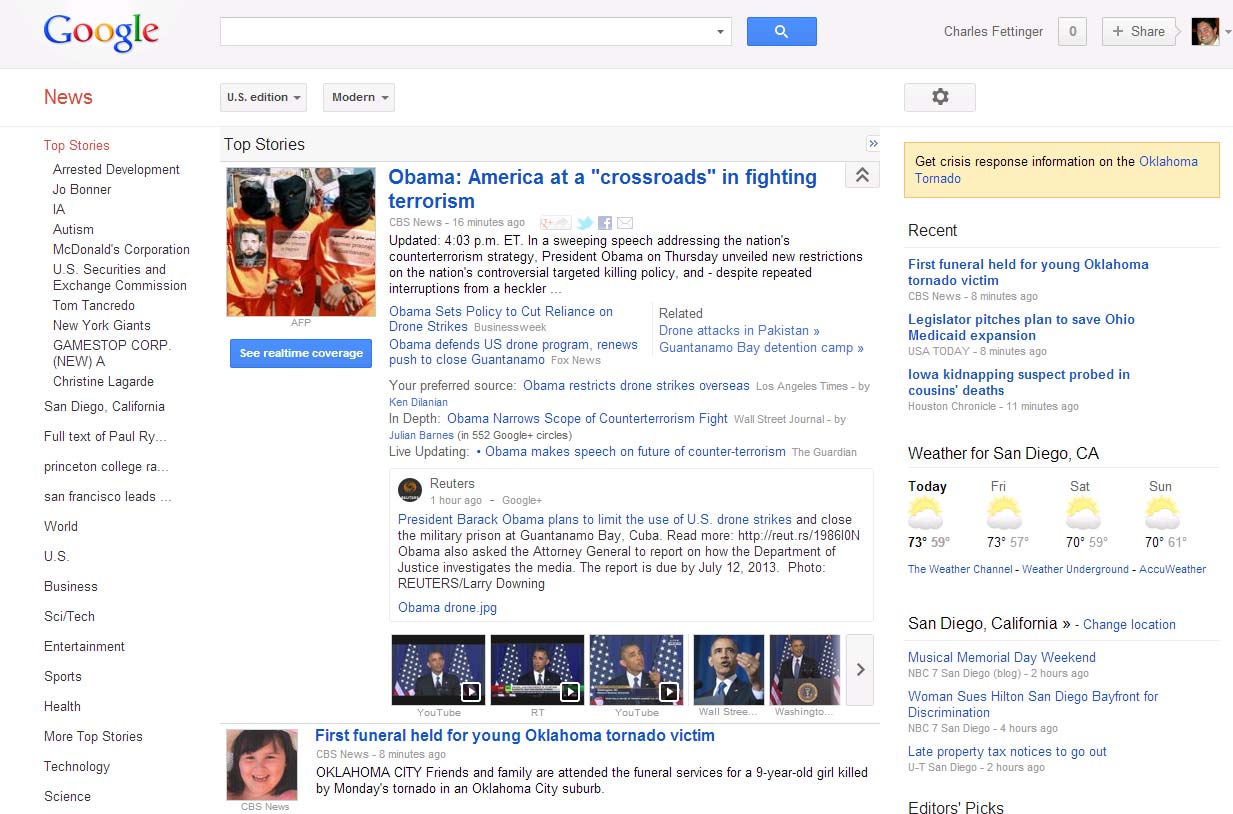The image depicts a Google page with several distinct elements:

- In the upper left corner, the Google logo is prominently displayed.
- To the right of the logo, there is a search bar with a magnifying glass icon inside a blue rectangle.
- Further right, the user's name, "Charles Feltinger," is shown, along with a square indicating they have zero notifications.

On the left side of the page, there are several categories and subcategories listed:
- The word "News" is clearly visible, with its subcategories including:
  - "Top Stories" highlighted in red, featuring articles like "Arrested Development Joe Bonner IA," "Autism McDonald's Corporation," "U.S. Securities and Exchange Commission," "Tom Tancredo," "New York Giants GameStop Corp," "San Diego, California," "Full Text of Paul Rye," and "Princeton College."
  - Other sections like "World," "U.S.," "Business," "Tech," "Entertainment," "Sports," "Health," "More Stories," "Technology," and "Science."

The main story on the page features an image of three men in orange jumpsuits, handcuffed, and wearing black masks. Beside this image, in bold blue text, is the headline: "Obama: America at a 'crossroads' in fighting terrorism."

To the right of the main story, the weather for San Diego, California, is displayed, showing sun and clouds.